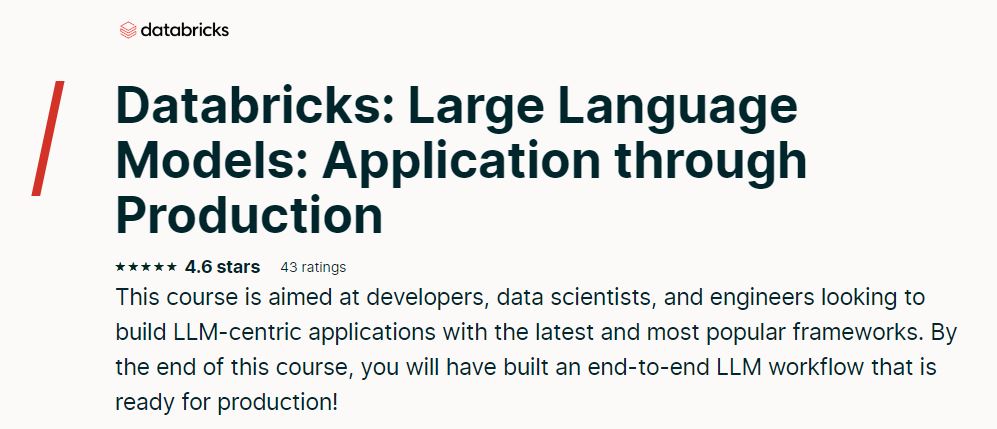This image features a detailed printout for a Databricks course titled "Databricks Large Language Models Application through Production," highlighted by a red, left-slanted line. At the top of the printout, the Databricks logo is prominently displayed in red, with "Databricks" written in bold, all lowercase letters. The course boasts an impressive rating of 4.6 out of 5 stars based on 43 reviews. This course specifically targets developers, data scientists, and engineers interested in constructing applications focused on large language models using the most current and popular frameworks. By the end of the course, participants will have the skills to build a comprehensive, production-ready large language model workflow. The course title is bolded for emphasis, while the remaining descriptive text is in regular font.